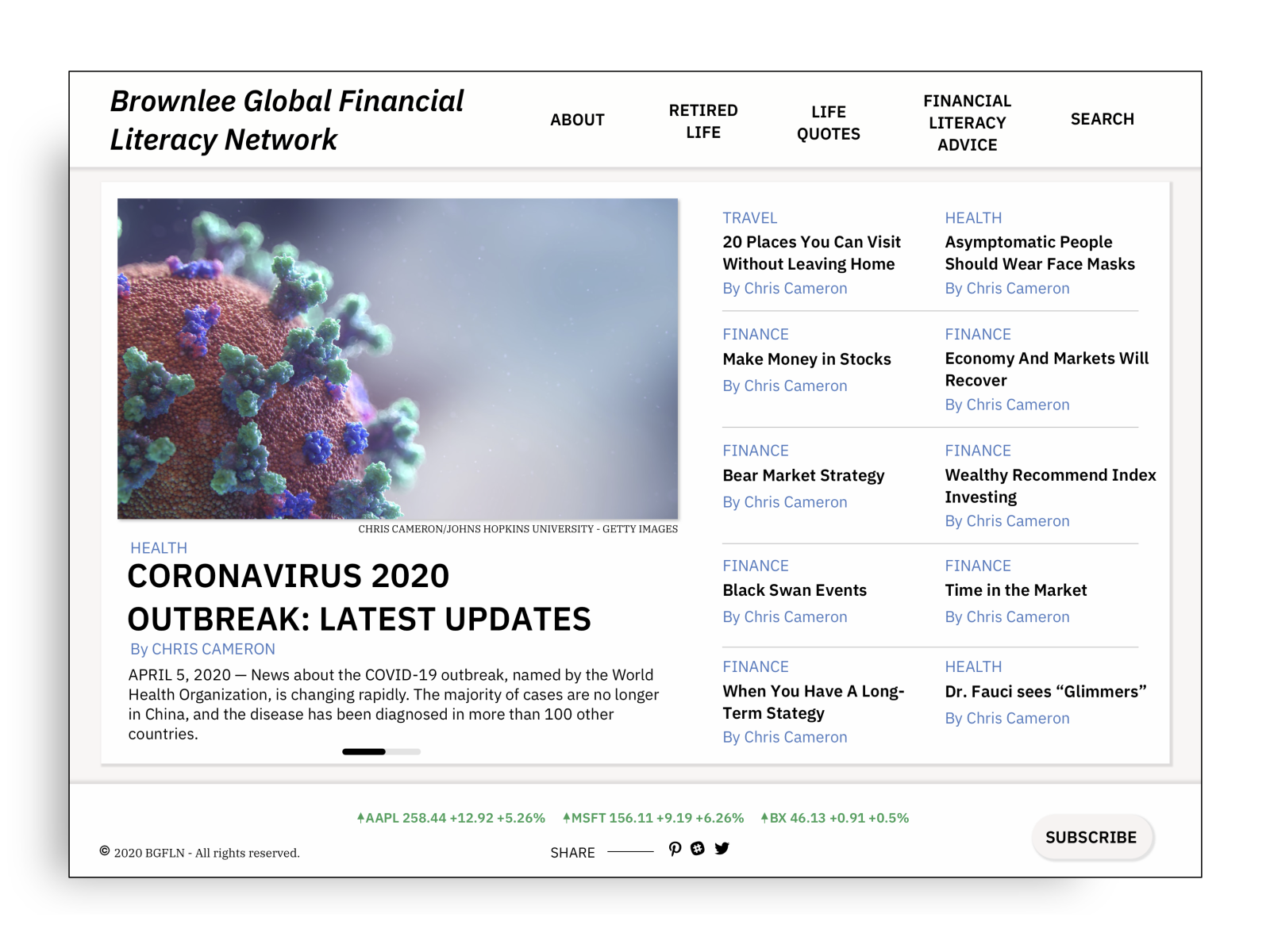This is a detailed caption for an image of a computer page showcasing a news and financial information website:

---

**Screenshot of a computer page from Brownlee Global Financial Literacy Network** 

In the top left corner, the website's name "Brownlee Global Financial Literacy Network" is displayed in black text. Spanning the top are several hyperlinks, including: "About," "Retired Life," "Life Quotes," "Financial Literacy," "Advice," and "Search."

Beneath this menu, on the left-hand side, there's a close-up image of the coronavirus. Below the image, a headline reads: "Coronavirus 2020 Outbreak Latest Updates by Chris Cameron." Dated April 5th, 2020, the news article discusses the rapidly changing information about the COVID-19 outbreak, noting that the majority of cases are no longer concentrated in China and have spread to over 100 other countries.

To the right of this article, there are two columns of news headlines under various categories. The first column includes:
- **Travel:** "20 Places You Can Visit Without Leaving Home"
- **Finance:** "Make Money in Stocks"
- **Finance:** "Bear Market Strategy"
- **Finance:** "Black Swan Events"
- **Finance:** "When You Have a Long-Term Strategy"

The second column features:
- **Health:** "Asymptomatic People Should Wear Face Masks"
- **Finance:** "Economy and Markets Will Recover"
- **Finance:** "Wealthy Recommend Index Investing"
- **Finance:** "Time in the Market"
- **Health:** "Dr. Fauci Sees Glimmers"

At the bottom of these columns, the byline, "By Chris Cameron," is shown. 

In the bottom right-hand corner of the page, there is a "Subscribe" button, along with share icons for Pinterest, Twitter, and another unidentified platform.

---

This caption provides a comprehensive overview of the elements present on the web page while maintaining clarity and detail.